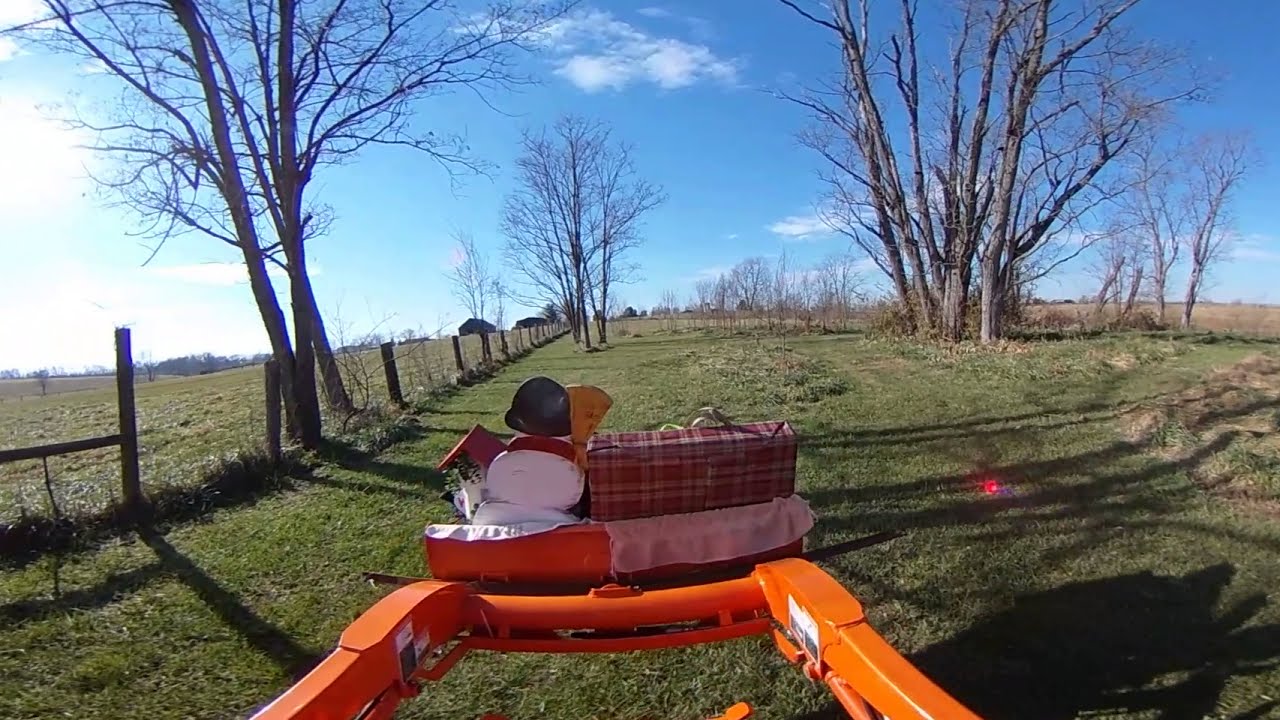This photograph captures a serene outdoor scene, possibly a park, garden, or farm field, covered with lush green grass and dotted with several dry, leafless trees, suggesting a fall setting. Dominating the foreground is the front part of an orange bulldozer or large wagon, partially obscured but filled with various household items, including a cushion, a teddy bear toy, and other miscellaneous objects. The scene is framed to the left by a fence, and the vivid blue sky overhead is scattered with white clouds, with shadows of trees and the fence casting across the right side of the field.